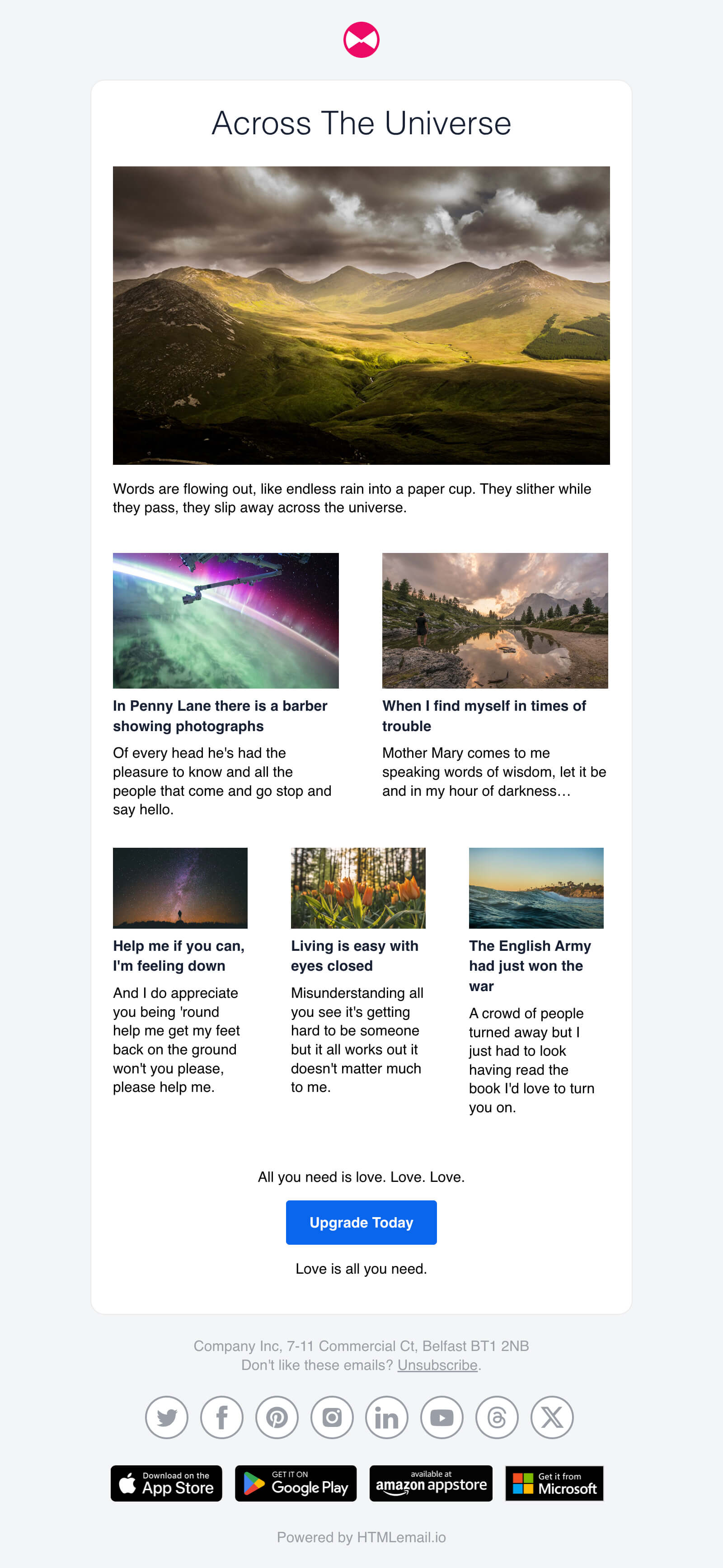This image features a collage incorporating text and various pictures. At the top, there is a prominent red and white circle. Beneath this, the text reads "Across the Universe." 

Below this title, there is an outdoor scene depicting a sky filled with white and gray clouds, with mountains looming in the background. The mountains display shades of yellow and green. The text below this image states, "Words are flowing out like endless rain into a paper cup, they slither while they pass, they slip away across the universe."

Further down, there are two separate pictures placed side by side. The left picture includes the text, "In Penny Lane there is a barber showing photographs of every head he's had the pleasure to know, and all the people that come and go, stop and say hello."

The right picture features a quote beginning with, "When I find myself in times of trouble, Mother Mary comes to me, speaking words of wisdom, let it be." The ending of this quote is cut off slightly, indicating that more text might be present beyond the visible portion.